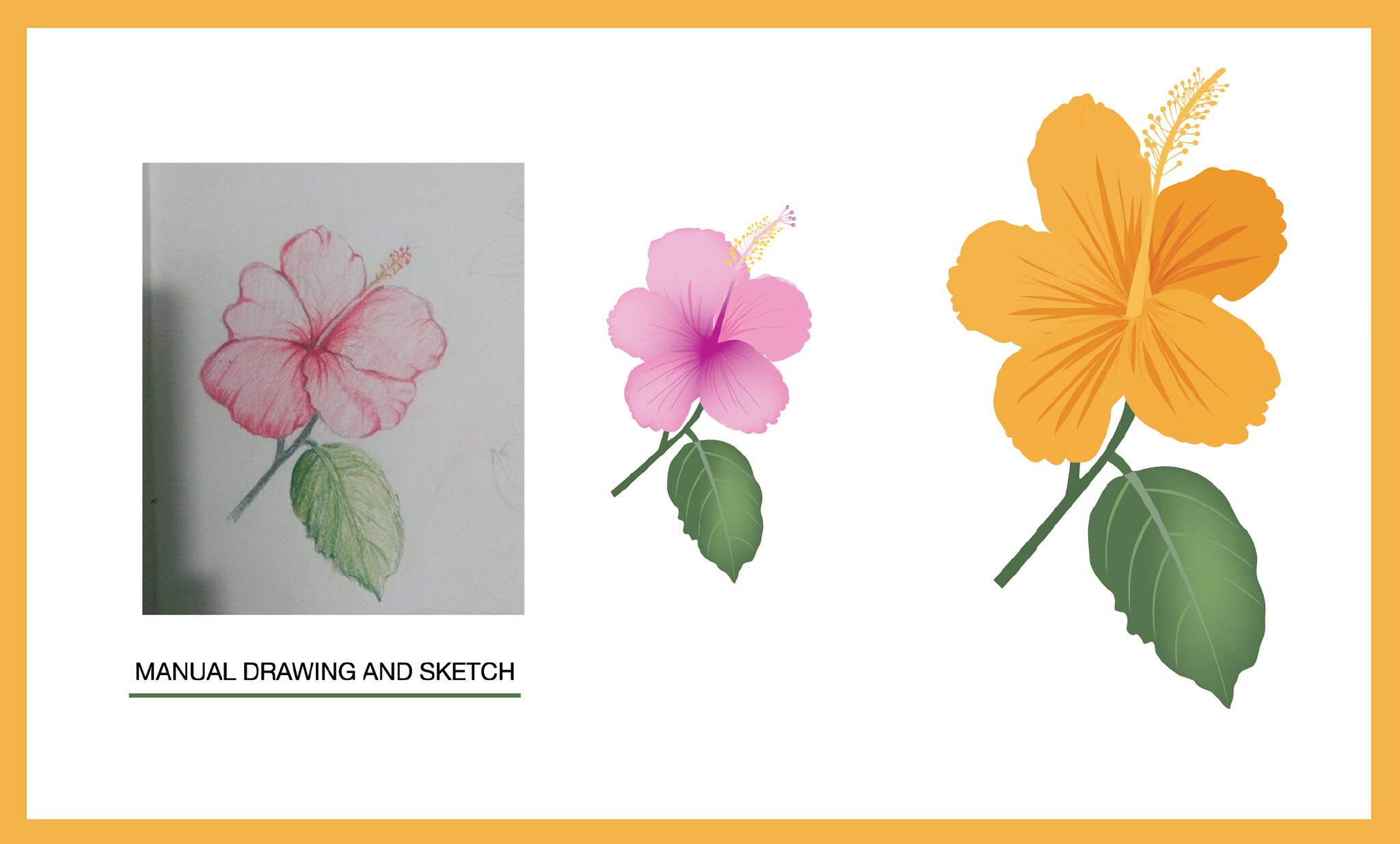This vibrant landscape-format illustration features a thin orange border framing a white background. On the left-hand side, an inset photograph showcases a delicate, hand-drawn sketch of a pink flower. Below this inset image, the caption reads "Manual Drawing and Sketch." Adjacent to the hand-drawn flower, an AI-generated or computer-generated illustration reveals an enhanced version of the same pink flower. The AI-rendered flower boasts brighter, more vivid colors and intricate detailing. To the far right, a larger, orange flower captures attention, mirroring the shape and design of the previous flowers. All three flowers are adorned with green stems and leaves, and their centers are detailed with fine pistils and stamens.